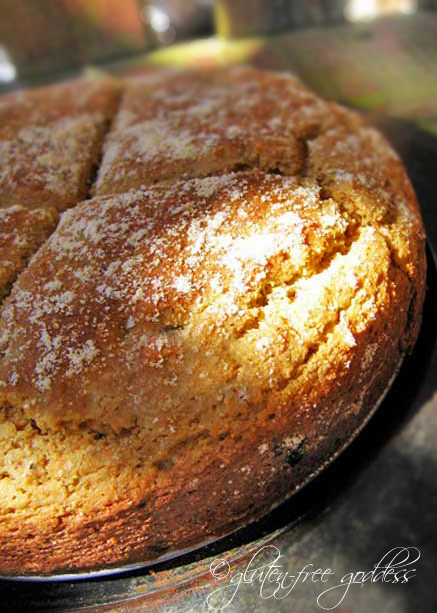This detailed color photograph showcases a close-up of a golden brown flaky pastry or bread, generously dusted with white powdered sugar. The bread, displayed in a silver pie tin, reveals a slice across the surface, adding to its rustic appeal. The tin rests on a gray stone table, with the background rendered into a soft blur. In the bottom right corner, a white cursive logo reads "gluten-free goddess," enhancing the artisanal charm of the image.